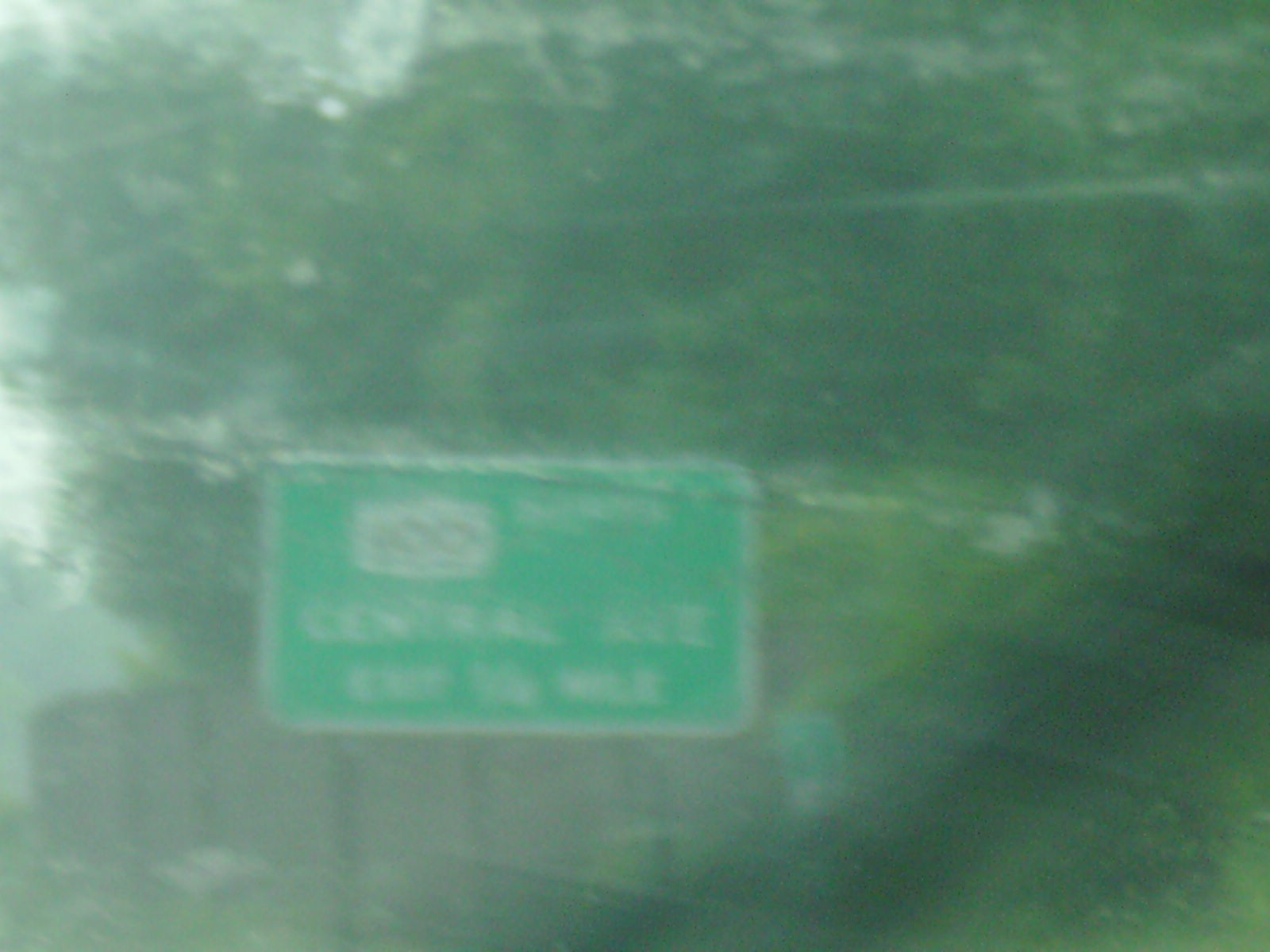The image appears to be taken from within a car, looking through the windshield. In the bottom right corner of the photo, there’s a somewhat indistinct, ghostly black object whose nature is difficult to determine. Through the slightly blurred glass, the viewer can observe the exterior environment. Prominently featured is a green road sign with the partially legible text "Central Avenue" and another piece of information regarding mileage at the bottom. Also visible on the sign is a white shield shape bearing some sort of number, supported by three poles. Behind the sign, there is a brown fence and another smaller green sign off to the side. In the background, green trees are noticeable, with the white sky peeking through in the top left corner of the image.